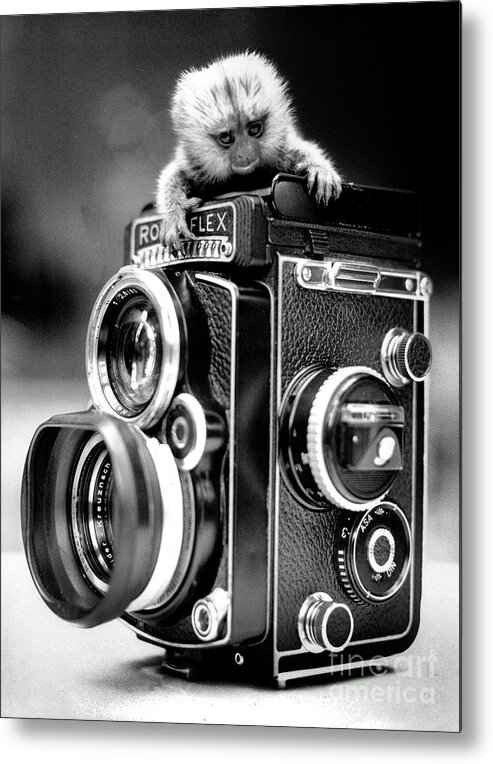This detailed black and white photograph features an old-fashioned, black camera with a bulky, vintage design. The camera is adorned with numerous knobs, dials, and two prominent lenses on the front. The camera is finished in a black leatherette and bears the partial inscription "R-O something flex," partially obscured by a small monkey's hand.

The focal point of the image is a tiny, fuzzy monkey perched atop the camera. The monkey has a circular head with light or white fur and distinct black rings around its eyes, giving it an owl-like appearance. Its eyes are light-colored, and it appears to be gazing down at the camera's body. The monkey is gripping the sides of the camera with its front legs, while its small, sharp nails are visible. The monkey’s expression is relaxed, and it shows no prominent ears.

The background of the image is blurred, creating a contrast that emphasizes the detailed textures of the monkey and the camera. The photograph also contains a transparent watermark in the bottom right corner that reads "Fine Art America."